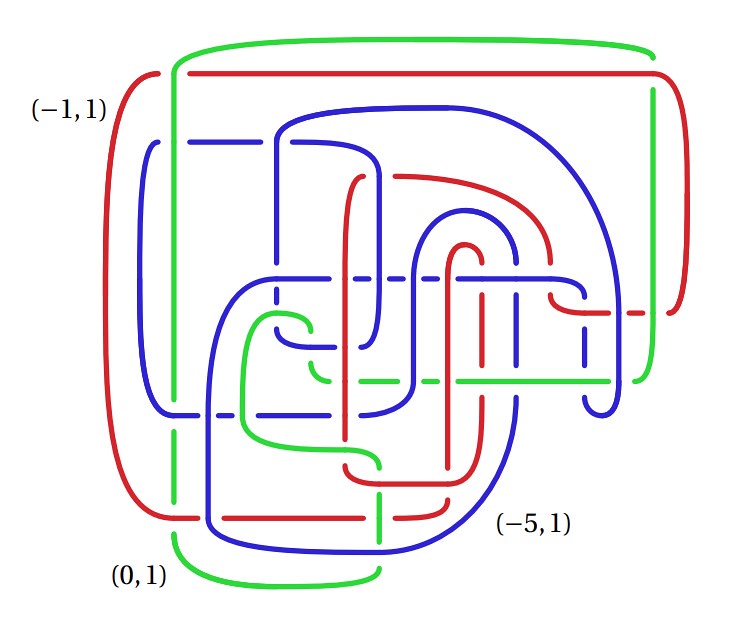This image features three distinctively colored lines—red, blue, and green—intricately interwoven and tangled against a pristine white background. In the upper left corner, the coordinates (-1, 1) are displayed, with the red line being proximate to this point. The bottom left shows coordinates (-0, 1), while near the bottom right corner, the coordinates (-5, 1) are present. These coordinates serve as positional markers within the image. 

The lines meander, crossing paths with one another in a complex pattern. Notably, rather than simply overlaying, when different colored lines intersect, there are deliberate breaks, creating a visually engaging and dynamic intersection. The lines form a series of square-like shapes, laid out in parallel and perpendicular orientations, interspersed with curving segments, particularly prominent with the blue line. There is no single geometric shape or definitive path; instead, the image is a harmonious mesh of line patterns that weave in and out, forming a chaotic yet mesmerizing web.